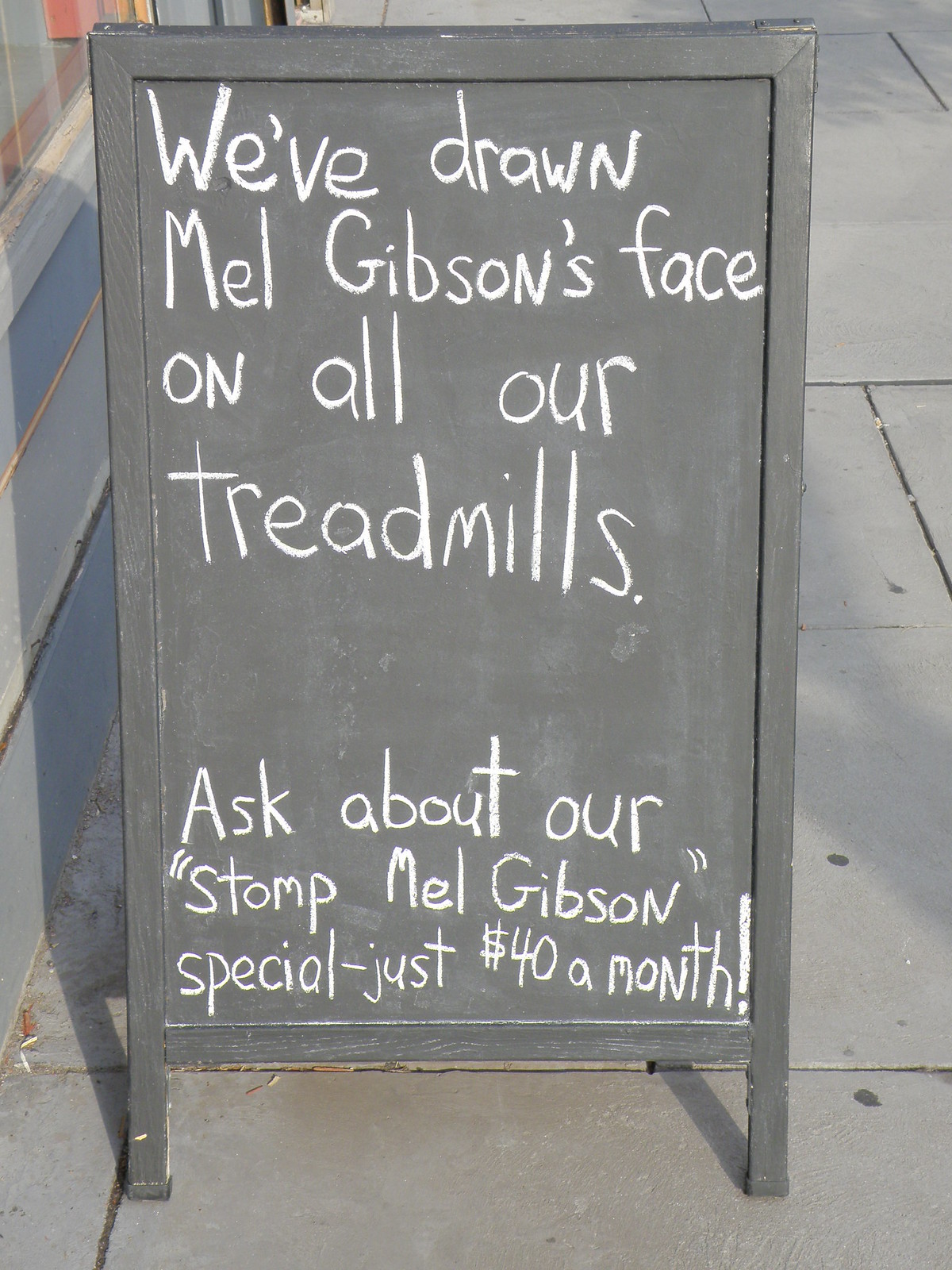The image depicts an outdoor scene featuring a wooden chalkboard sign with short legs placed on a concrete sidewalk. The sign has a black chalkboard area with white chalk writing, displayed against what appears to be a background of light gray concrete and the lower parts of a building, including the bottom edge of a window to the left. The chalkboard content advertises a gym promotion and reads: "We’ve drawn Mel Gibson’s face on all our treadmills," followed by "Ask about our 'Stomp Mel Gibson' special - just $40 a month!" The sign casts a shadow to the left that stretches up a wall featuring three slightly diagonal gray stripes. The intended humor appears to be a draw for potential customers to inquire about the unique and creatively named gym offer.